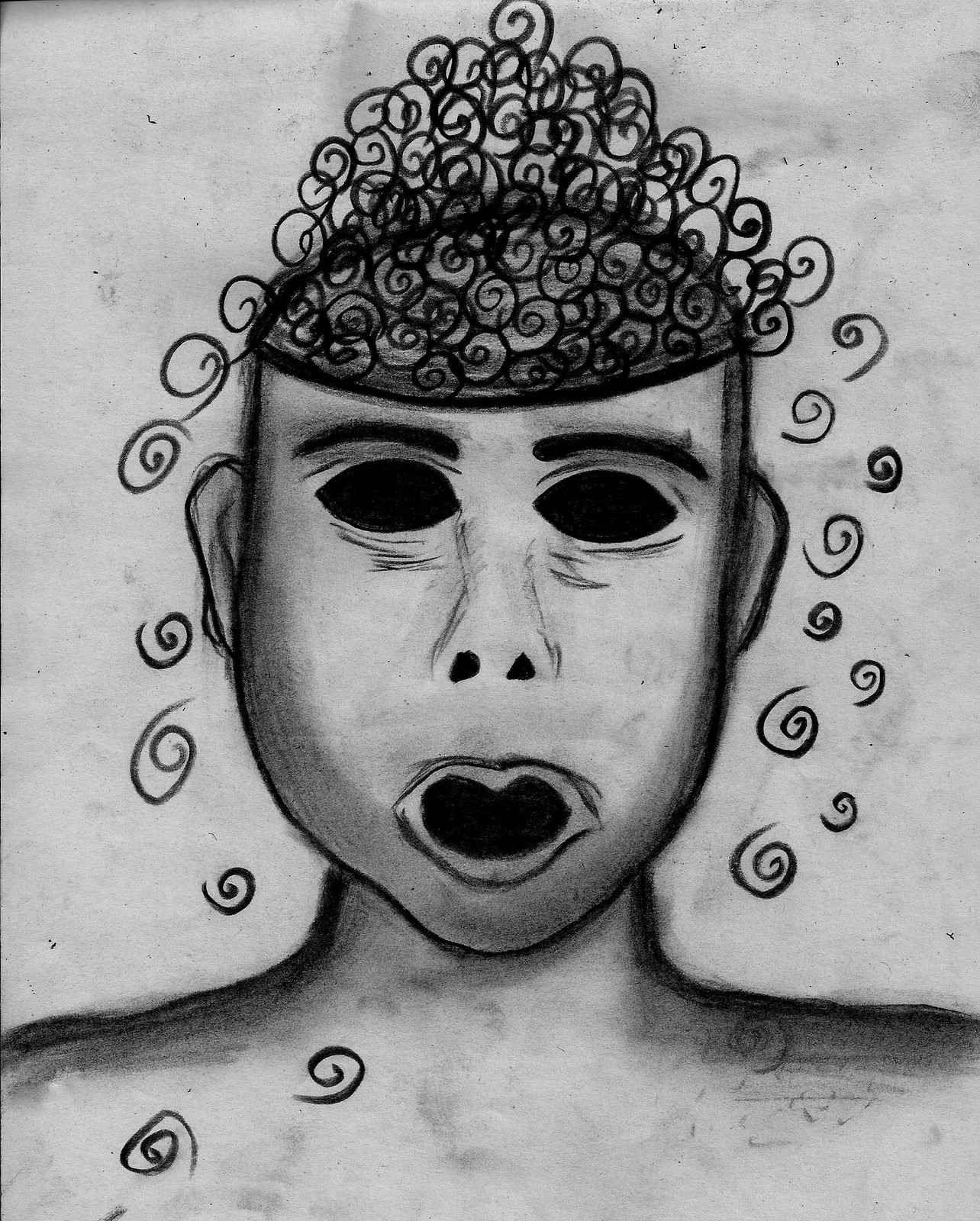The image is a black-and-white scan of a detailed pencil or charcoal artwork on gray paper. It depicts a male-like figure from the shoulders up with intensely expressive features. The eyes are hollow, black voids without eyeballs, creating a haunting stare, and the mouth is wide open, also appearing void-like. Thick eyebrows add to the intense expression. The shoulders are heavily shaded in black, enhancing the figure's somber and eerie appearance. The most striking element is the top of the head, which seems to have been cut straight off, with a cascade of swirly, curly lines falling from where the scalp would be, as if suggesting hair or perhaps a more abstract, chaotic emission from the head. The overall thick, varied lines and shadows give a profound sense of depth and texture to the artwork.